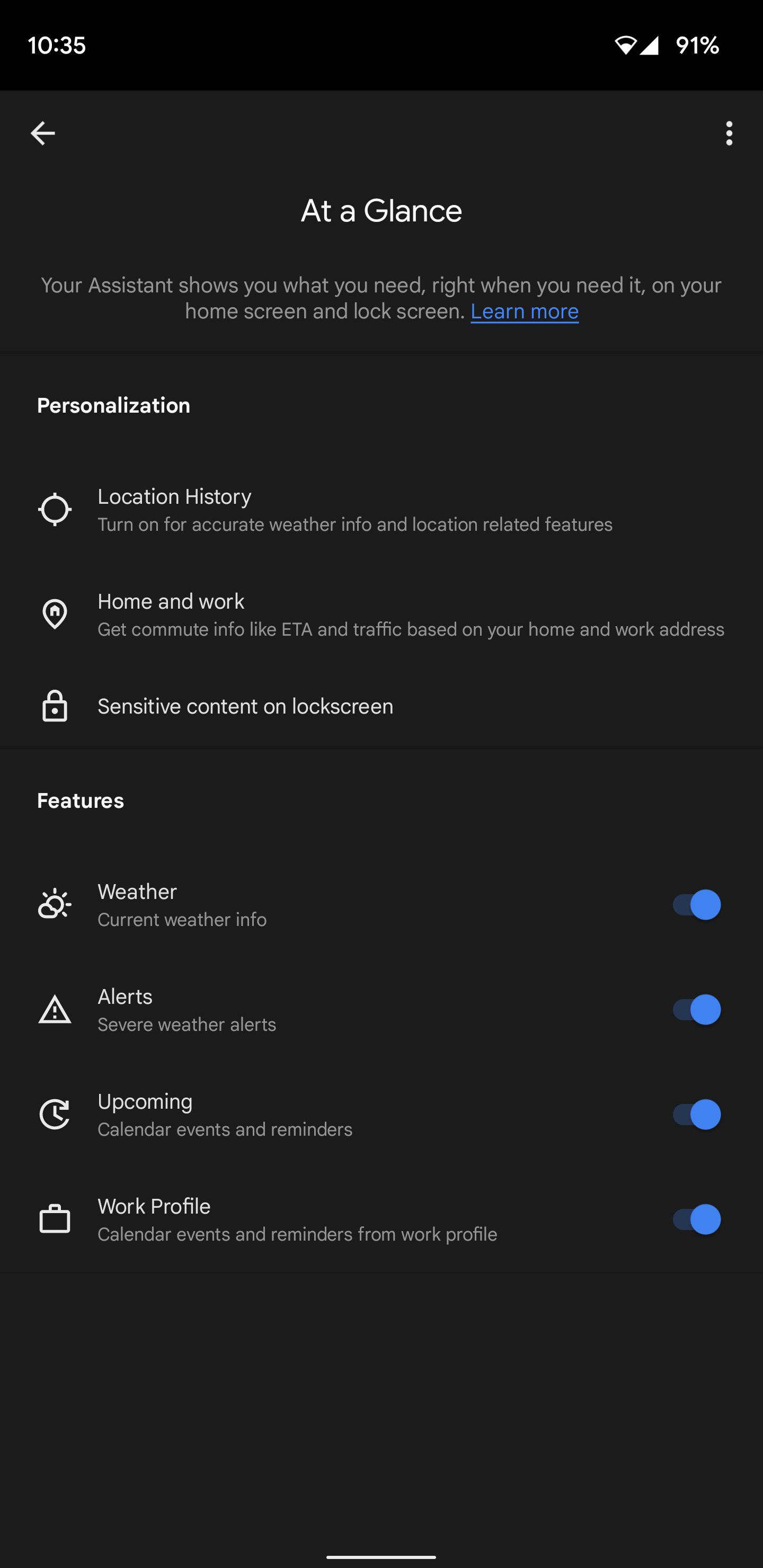On a sleek black background, the image showcases a seamless interface with a header reading "1035" and "91%," featuring a left arrow icon. Just below, there are three vertical dots indicating more options. The prominent section titled "At a Glance" offers quick, personalized insights, smartly assisted for optimal convenience.

This interface allows customization and personalization, including notable elements such as location history—highlighted for quick access. Essential information regarding home and work locations is visibly listed. The display also includes settings for sensitive content on the lock screen, ensuring privacy and discretion.

Noteworthy features include a detailed weather forecast section, featuring toggle bars for receiving current weather info and service alerts. There are also toggles for upcoming weather alerts, enabling proactive updates. Calendar events and reminders are neatly organized, with toggle options available for both personal and work profiles, ensuring streamlined task management.

For more information or to delve deeper into customization options, a "Learn More" link is provided in blue, guiding users towards expanded functionalities and additional settings.